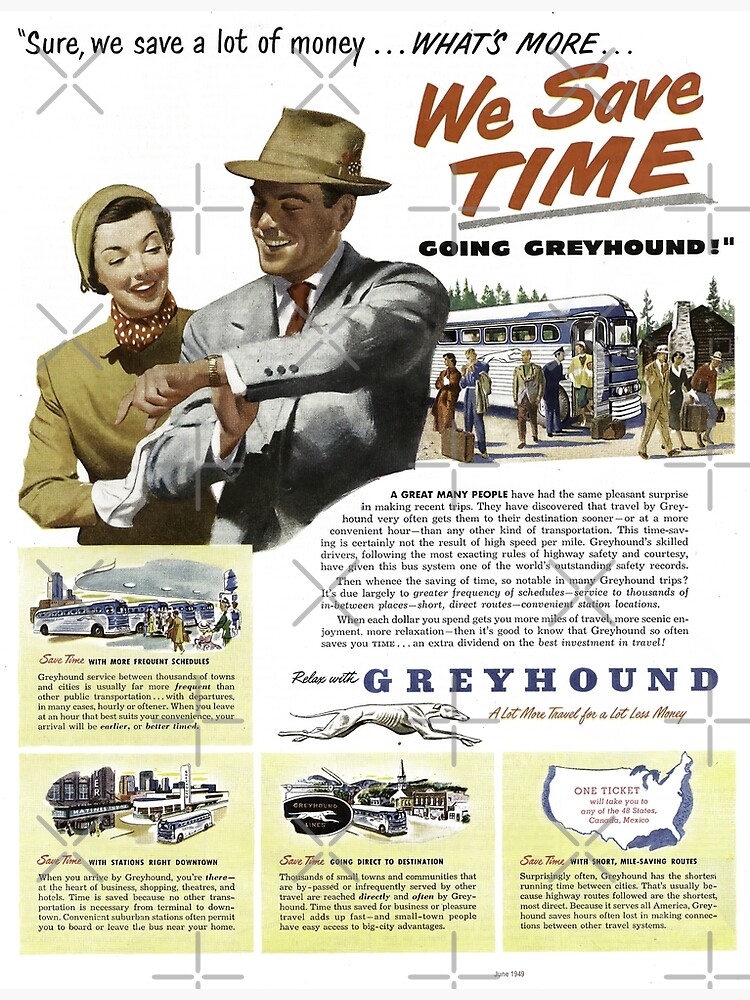This vintage advertisement for the United States Greyhound bus service, likely from the 1950s, prominently features a well-dressed couple in business attire with joyous expressions. The man, holding up his wristwatch, underscores the ad's headline: "Sure, we save a lot of money. What's more, we save time. Going Greyhound." The primary colors of the ad—yellow, red, blue, and black text—enhance its vibrant appeal.

In the top left corner, the couple stands beside the bold red font that emphasizes the time-saving aspect of Greyhound travel. Below this, a Greyhound bus is depicted, with passengers disembarking, suggesting they have reached their destination. The bottom part of the ad is populated with four yellow squares highlighting features like "stations right downtown," "direct to destination," and "short routes on one ticket." Additional text extols the timely and convenient travel advantages of Greyhound over other modes of transportation. To the center, a bus is shown against a backdrop with a cityscape on the left and a map of the United States on the bottom right, visually reinforcing the widespread network and accessibility of Greyhound buses.